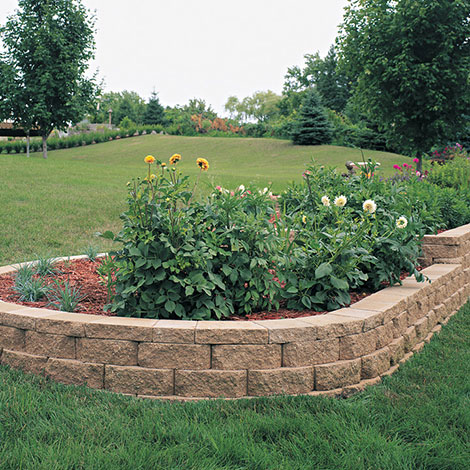This outdoor daylight photograph captures a large, well-maintained green lawn extending into the background, where it gently rises up a short hill. Prominently featured in the foreground is a low wall constructed of brown stone bricks, about three bricks high, encircling a flowerbed filled with red mulch. Within this bricked-off area, vibrant foliage showcases a mix of dark green leaves and an array of flowers, including small yellow blooms more on the left, white flowers on the right, and a scattering of pink and purple flowers towards the middle right. 

The lawn in front of the wall stretches out flat, displaying well-kept grass. Toward the upper left and upper right corners of the image, several bushes and trees frame the scene, providing a natural border. In the far left background, a hedge marks the edge of the lawn, beyond which a mix of taller, more intermixed trees can be seen. These trees have an orange hue, although details are indistinct. Farther to the back, the sky looms overcast and gray, without distinct clouds, casting a diffuse light over the entire garden.